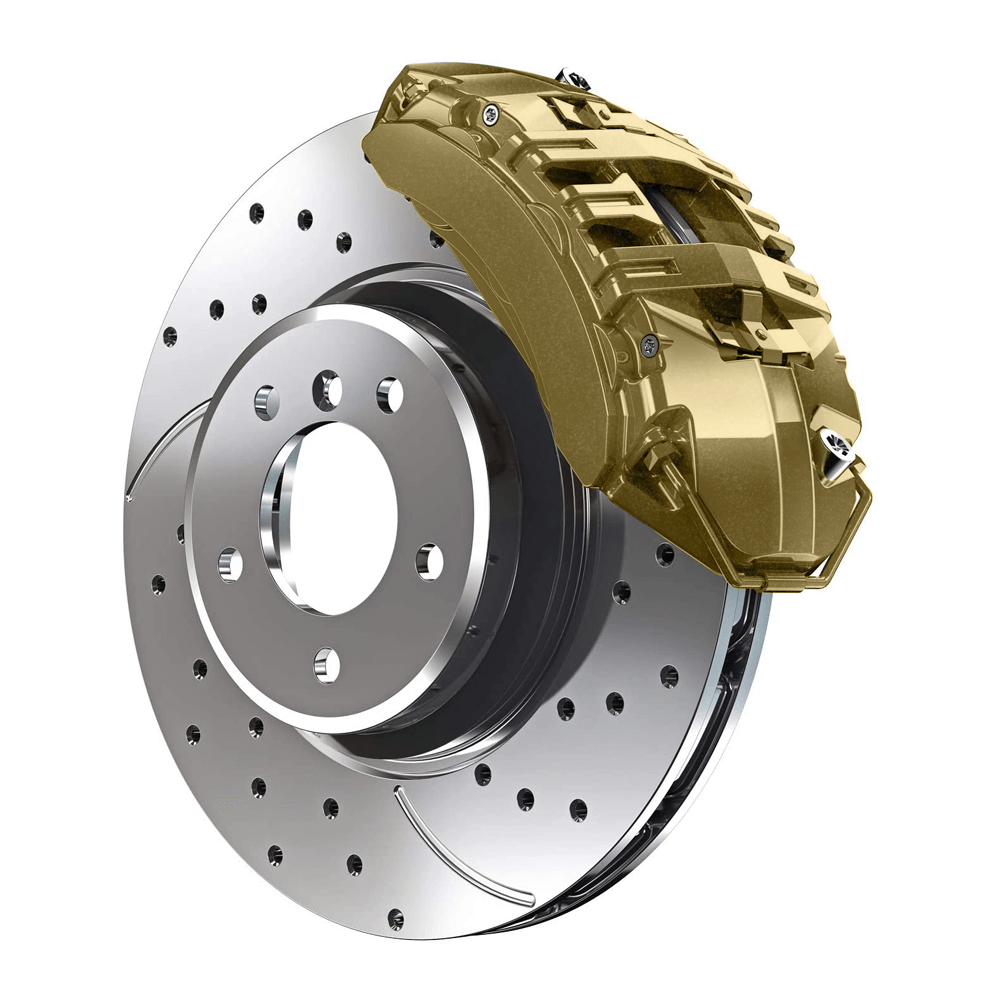This vertical, borderless image appears to be a highly detailed 3D color illustration or photograph of a high-performance car disc brake system, presented on a white background. The silver brake disc, seemingly made of stainless steel, features a series of strategically placed holes around its edge for cooling purposes. Its surface is smooth, intended for the brake pads to clamp onto it. At the center of the disc, multiple holes are designed for various lug nut configurations, likely to accommodate different car models with a five-lug setup. Surrounding the central hub, the disc showcases a sophisticated design with swirling patterns and black insertions, possibly for added structural integrity or aesthetic appeal. Resting on the top portion of the disc is the gold-colored brake caliper, a semi-circular housing that contains the brake pads. This caliper perfectly follows the curvature of the disc, suggesting a precise and close fit necessary for effective braking. The overall image appears to float due to its white background, emphasizing the detailed, product-photography style of the illustration.